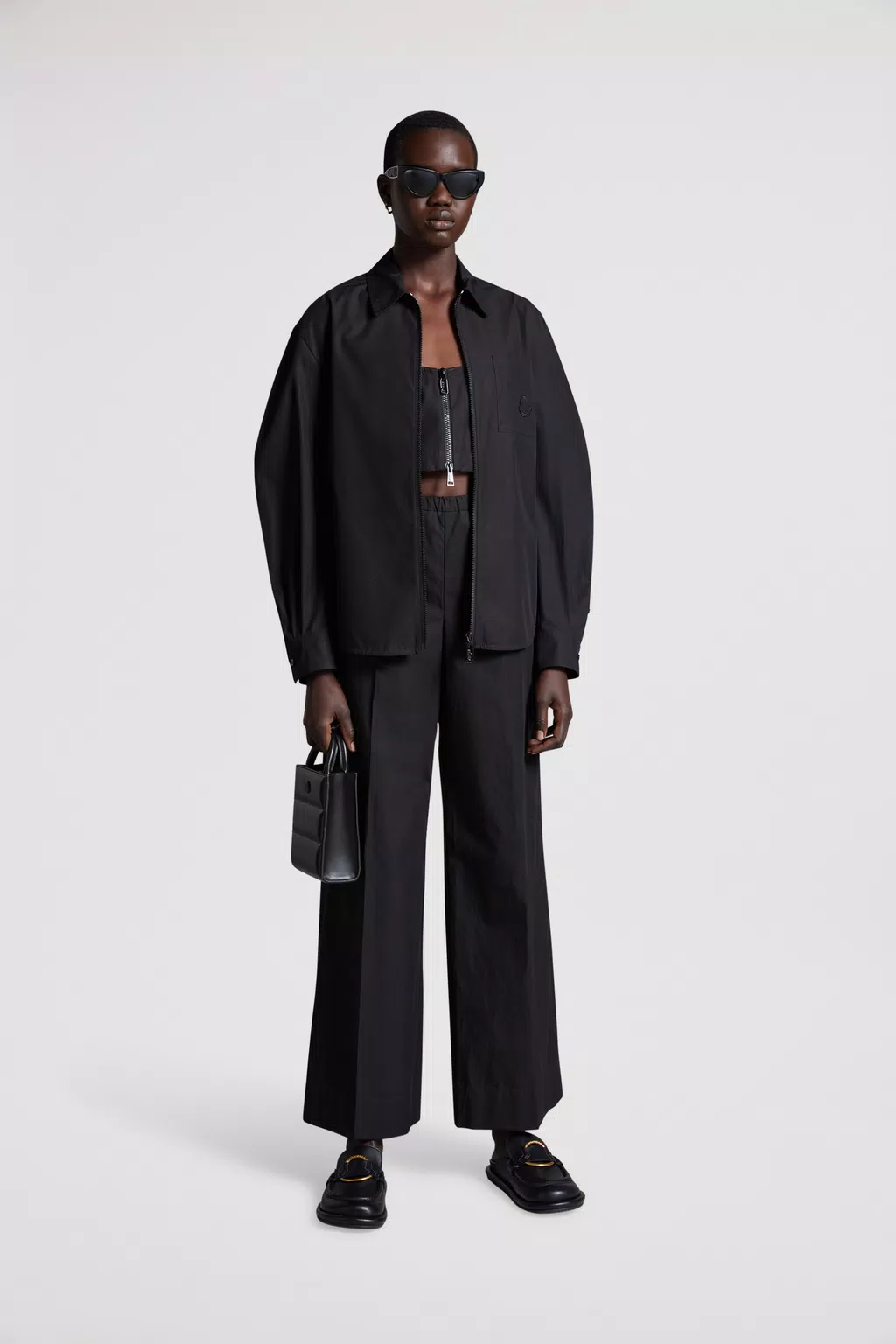In this vertically-oriented portrait, a striking young black woman stands confidently against a gray background that seamlessly blends the wall and floor. Her very short, cropped hair is complemented by large black sunglasses and small earrings, primarily visible on her right ear. She dons a black ensemble consisting of a stylish jacket with a zipper and wide-leg pants, alongside a half-shirt, or crop top, which reveals a glimpse of her abdomen. She clutches a small black bag in her right hand, with her arms hanging straight down by her sides. Her footwear consists of wide, black loafer-style shoes adorned with large golden buckles, adding a touch of elegance to her modern, minimalist outfit. With a neutral expression, she gazes directly at the camera, exuding an aura that is both poised and fashion-forward, suitable for a high-end fashion catalogue or a sophisticated high street collection.